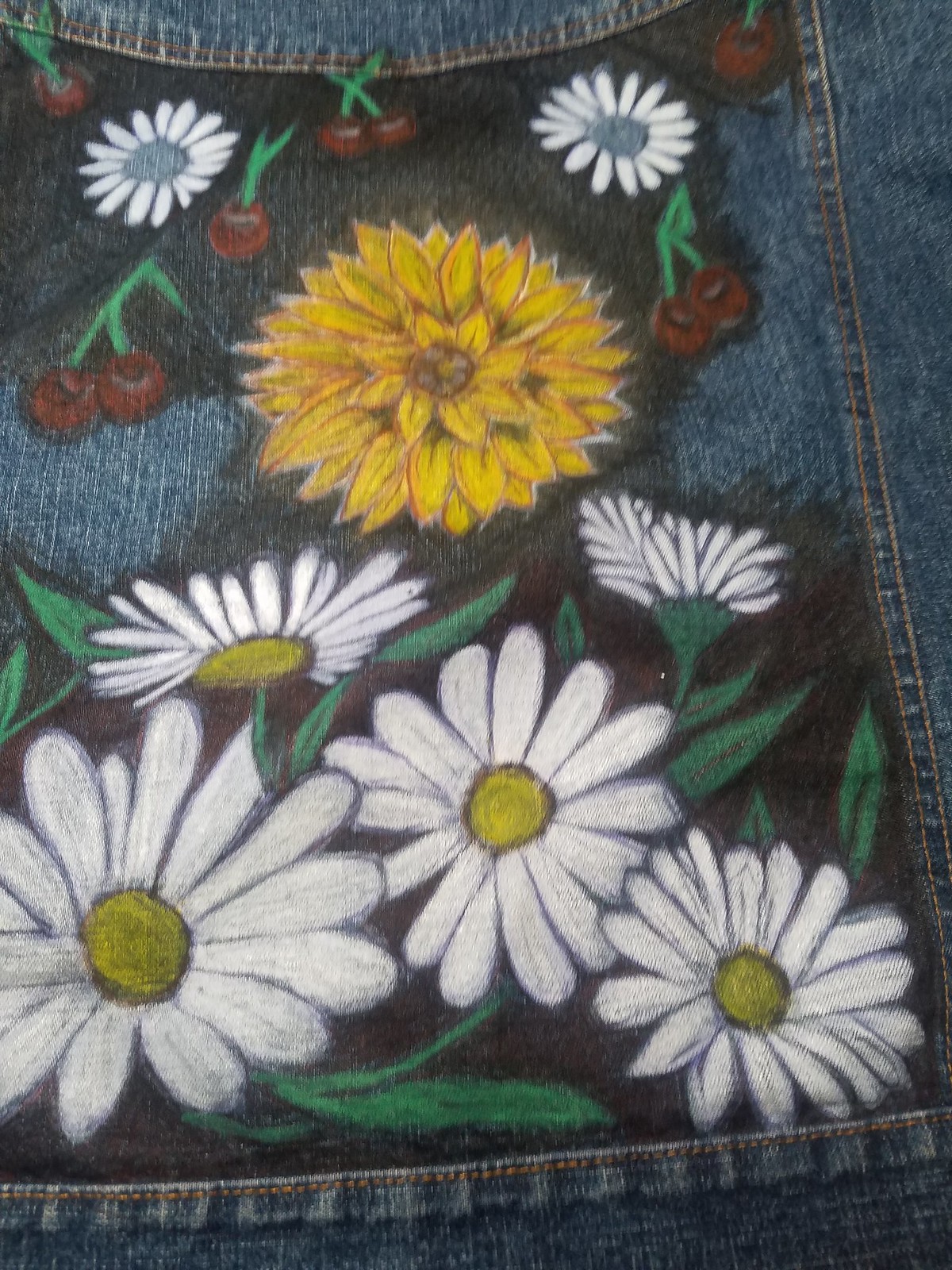The image is a highly detailed, hand-painted design on medium blue denim, likely part of a jean jacket or a pocket. The background mimics the textured fibers of denim with shaded blue hues. The design is accentuated with coppery stitching along the seams.

Centrally, a prominent yellow chrysanthemum with orange-outlined petals and a light beige center stands out. Surrounding this are various flowers and vibrant cherries. There are delicate white-petaled daisies with yellow centers, scattered predominantly towards the bottom and some with blue centers near the top. Two distinct groups of paired red cherries on green stems flank the main flower, with additional single cherries interspersed around the design.

The entire background behind the floral and fruit elements is painted black, making the colors pop vividly. Small green leaves are integrated throughout the composition, adding to the lush and intricate aesthetic of the artwork.